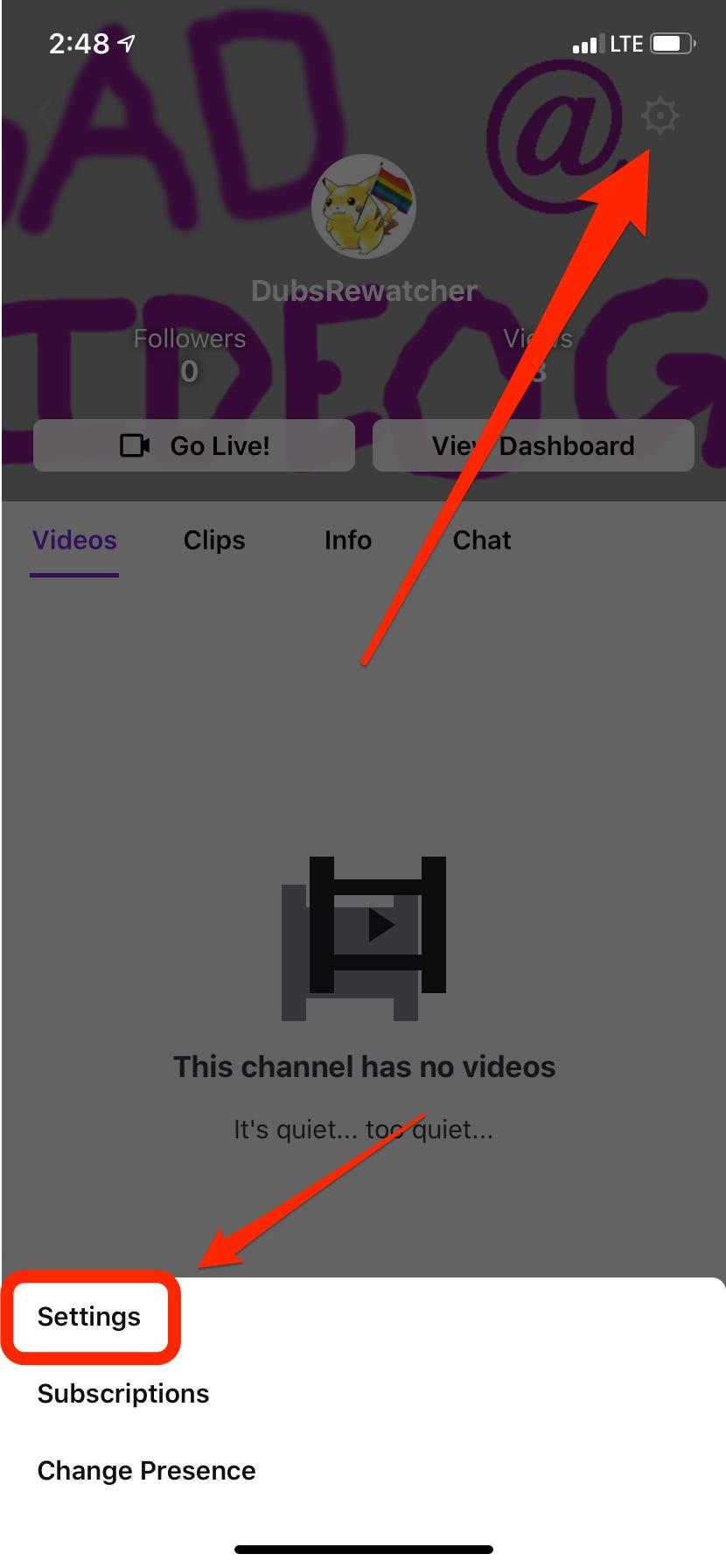This image is a detailed, annotated screenshot of a mobile phone displaying a YouTube channel's settings page. The mobile phone's status bar at the top shows a white font indicating the time as 2:48, a location sharing icon on the upper left, 3 out of 4 bars of LTE on the upper right, and a battery life at 75%. The screenshot includes a gray filter overlay and captures the channel settings, highlighted by various photoshopped red arrows for emphasis. 

The channel settings screen shows a blue text banner at the top, which seems to be crudely designed using Paint Shop software. Below the banner is the channel’s profile picture, which features a Pikachu with a gay pride flag, all set within a white circle. The channel name displayed is "Dubs Rewatcher," which currently has zero subscribers and three visits. A red arrow on the upper right points at a gear icon, indicating the entrance to further settings. Another red arrow at the bottom highlights the black text labeled "Settings."